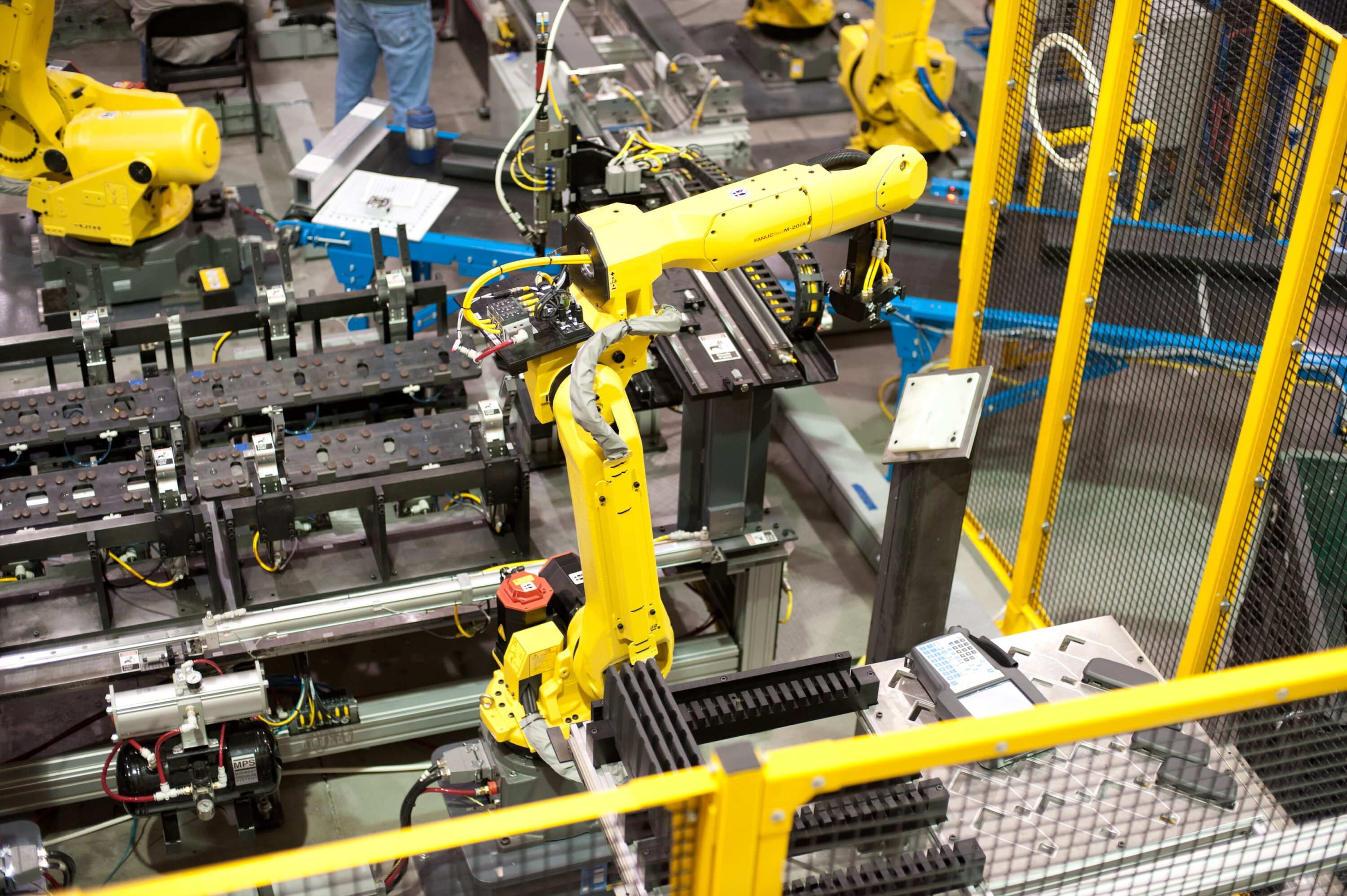In this vibrant factory scene, a network of robotic arms orchestrates a complex assembly line. Dominating the center of the image is a prominent yellow mechanical arm, characterized by its rectangular segments—one standing upright and another extending horizontally to the right. The robotic arm's structure includes a circuit board adorned with intricate red and yellow cabling, and a black control mechanism attached to its lower arm. Surrounding this main arm are additional yellow robotic arms, hinting at a synchronized manufacturing process.

Towards the upper left of the image, a worker's legs clad in blue jeans are partially visible, indicating human presence amidst the automated environment. Nearby, another individual appears to be seated on a black metal chair, identifiable only by their gray shirt. Above these human figures runs a blue and yellow conveyor belt, currently stationary, bearing black cylindrical objects.

In the foreground, vertical supports with a black grate serve as protective barriers for the robots. The factory space is filled with an array of black metal objects on racks and various mechanical components, contributing to the industrious atmosphere of this high-tech manufacturing facility. The overall impression is one of precision and efficiency, with both human and robotic elements contributing to the production process.